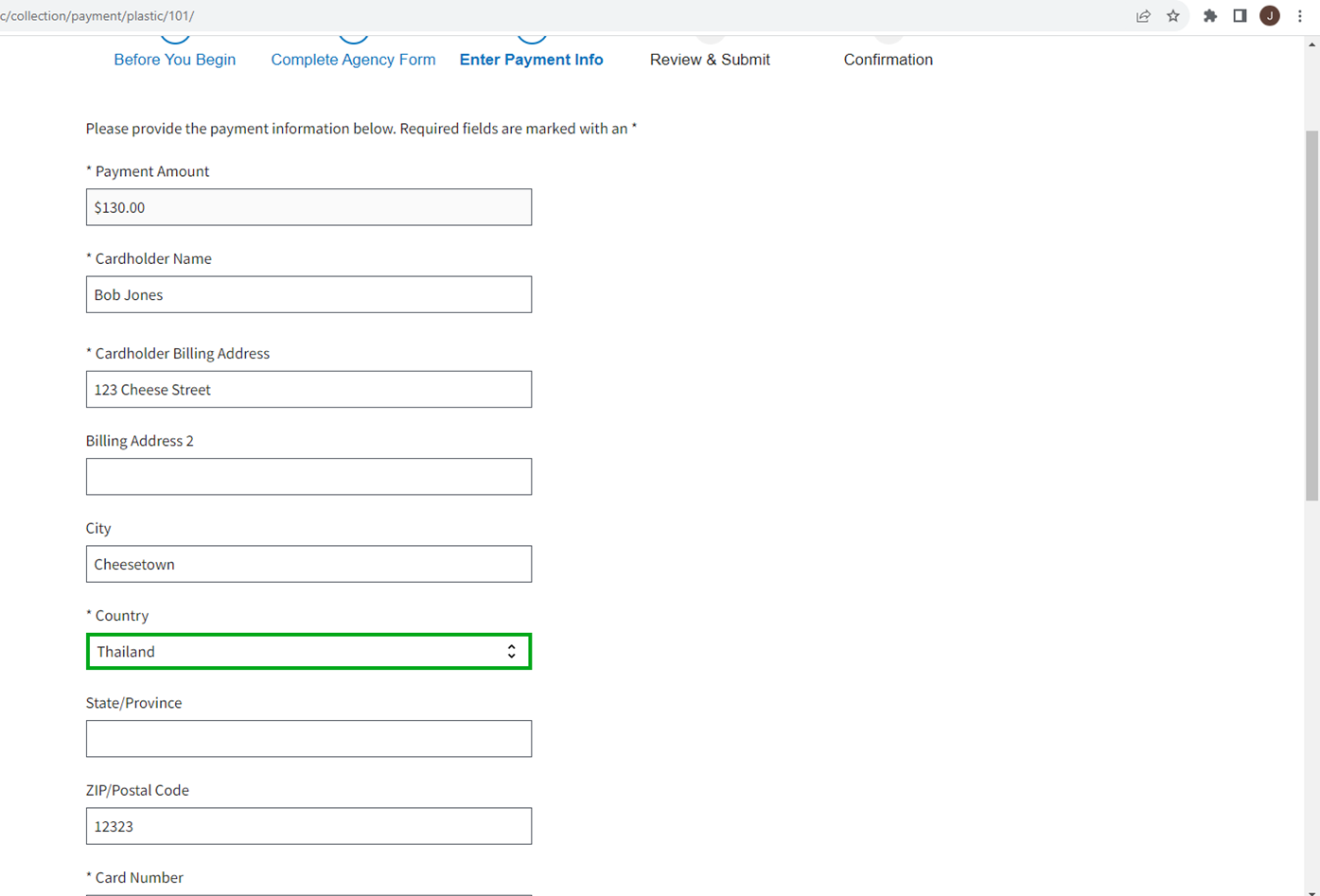The image depicts a payment page on a website, likely used for purchasing an item or paying a bill. The page's layout includes several key elements:

- At the very top, a light blue banner spans the width of the page. Within the address bar, it shows a URL that reads something like "collection/payment/plastic/101/". On the far right of this banner, there is a bookmarking star icon followed by an unclear symbol, and a menu icon consisting of three vertical dots.

- Below this banner, the background is predominantly white. The main section of the page is organized into a five-step process, displayed as blue text with circles above each step to indicate progress. The steps are:
  1. **Before You Begin**
  2. **Complete Agency Form**
  3. **Enter Payment Info** (This step is highlighted in a darker blue, indicating the current step)
  4. **Review and Submit**
  5. **Confirmation**

- At the top of the main content area, in black text, it instructs users to "Please provide the payment information below; required fields are marked with an asterisk."

- Following this instruction, several form fields are presented:
  - **Payment Amount**: Highlighted in light blue with "$130" inside.
  - **Name**: The name "Bob Jones" displayed in black ink within a white rectangle.
  - **Cardholder's Billing Address**: The address section with several sub-fields including:
    - **City**: Displays "Cheese Town."
    - **Country**: Highlighted in green.
    - Further fields for **State/Province**, **ZIP Code**, and **Card Number** are also present but not filled in within the description.

The visible content indicates a partial view of the page, as it appears to be scrolled down, cutting off the top of the circles representing the steps.